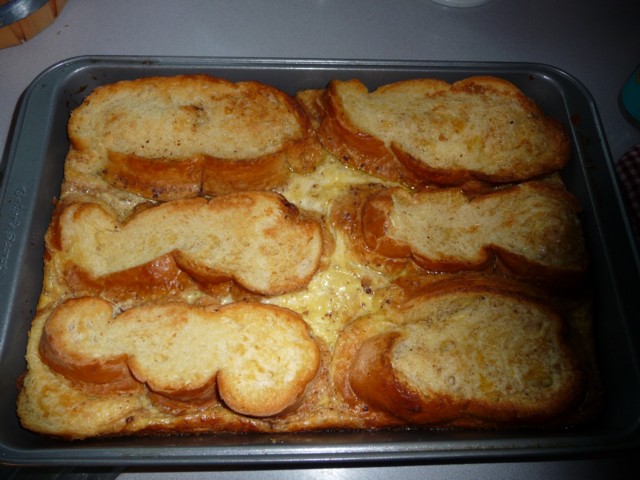The image depicts a large, dark gray metal baking pan with slightly raised edges, and a few spots of rust. The pan contains six pieces of variously sized bread that have been baked and somewhat toasted, displaying a golden brown surface with a white, buttery sheen. The bread sits atop a layer of melted cheese, giving it a gooey appearance, suggestive of being part of a lasagna-like dish. The crusts of the bread are notably brown, adding contrast to the composition. The baking pan rests on a light gray or bluish-gray countertop, with a small portion of an oven mitt visible on the right side. In the upper left corner, there’s a hint of a wooden circle and a silver object peeking into the frame.